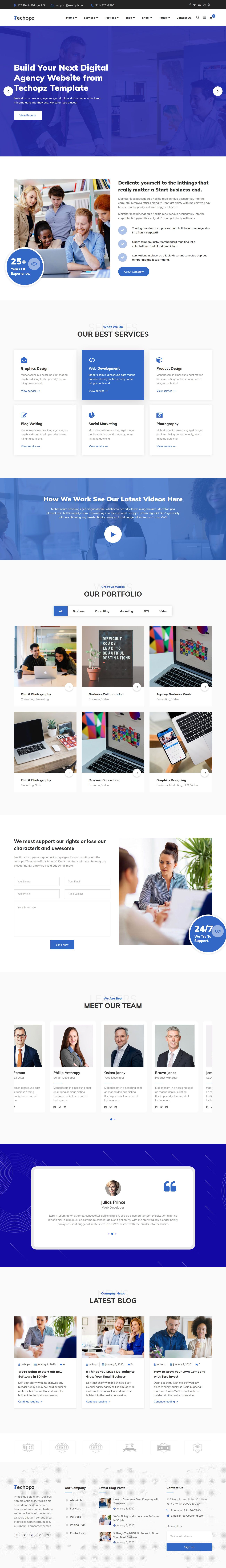**Descriptive Caption:**

This image is a vertically oriented, highly cluttered webpage screenshot that is challenging to decipher due to its distorted and compressed presentation. At the very top, a long black bar is visible, followed immediately by a white bar containing several unreadable black text links. Beneath this, a large blue bar with faint background watermarks features a person leaning over a table. This section contains some white text elements, including a clickable white bar with blue text.

Immediately below this, a distorted image depicts four or five people huddled over a laptop in what appears to be an office. Two individuals, both in blue shirts, appear to be Caucasian. To the lower left of this image is a blue oval with white text, and to the right is black text along with a long blue clickable oval.

Next, there are two rows of clickable choice boxes—each box containing unreadable text—situated within a faint gray box, with black text above the center of it. The middle box in the top row is highlighted in blue, indicating a selection. Further down, there's another long blue bar with faint background imagery of people and white text.

Following this section, a set of two rows with three pictures each is seen. In the top row, the leftmost image shows two individuals looking at a laptop, the middle image features a digitally created black box with white text and a plant, and the rightmost image displays another laptop. In the bottom row, the leftmost image is indiscernible, the middle replicates the laptop image from above, and the rightmost depicts a laptop, keyboard, and a smartphone.

Below these images, two text boxes and a clickable blue bar with black text and gray text above it are present. To the right, a rectangular image shows a Caucasian woman in a blue shirt, with another Caucasian woman partly visible, wearing a white shirt in front of a laptop with a green plant.

Further down, four pictures of people in business attire—three men and one woman—are aligned, accompanied by gray, unreadable text. Below this, another long blue bar contains a white box with unreadable text.

The final section includes three long, rectangular images that are challenging to discern. The leftmost contains a woman in a blue shirt, seemingly identical to an earlier image, while the middle depicts two Caucasians in light and dark blue shirts in front of a laptop. The rightmost features a man in a blue shirt and a woman with black hair in a white shirt by a laptop. Unreadable black text is found beneath this section. 

At the image's very bottom, a gray box with faint, unreadable black text is present. In the far lower right corner, a blue bar is visible and seems to be clickable.